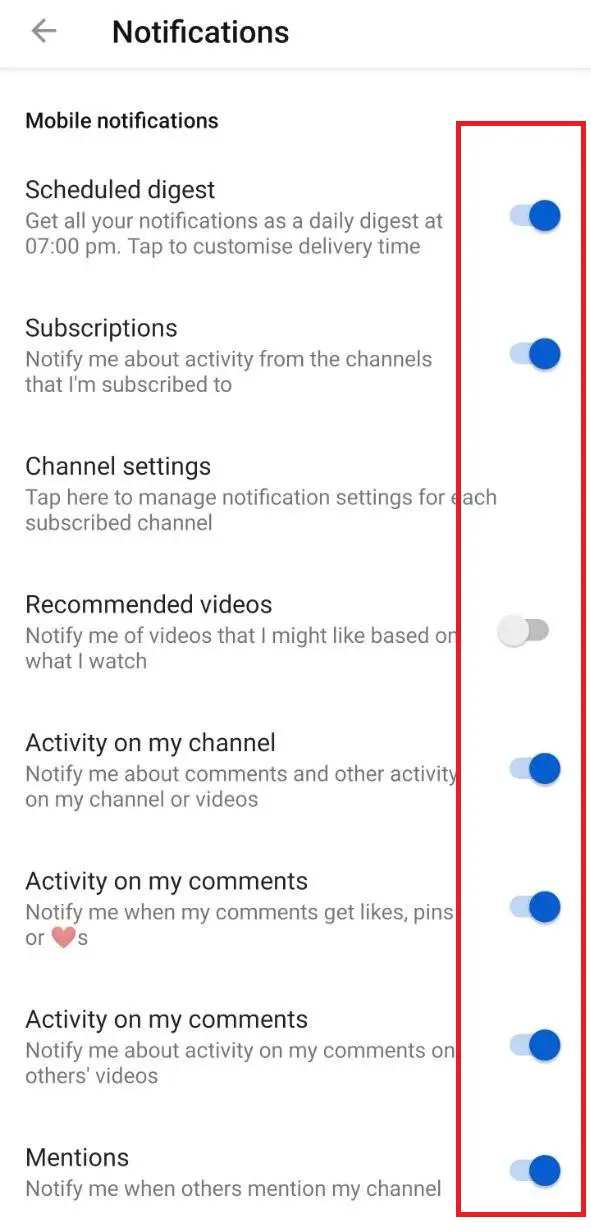This vertical image, likely a screenshot from a smart device, features a user interface for managing notification settings. The image predominantly presents a white background, with distinct sections separated by gray lines. 

In the top-left corner, a black arrow points left, next to the bold text "Notifications." Below, the section titled "Mobile Notifications" is indicated with a smaller yet bold font. This area contains several options:

- **Schedule Digest**: Get all your notifications as a daily digest at 7 p.m. (Blue toggle switch indicating ON)
- **Subscriptions**: Notify me about my activity from the channels that I'm subscribed to. (Blue toggle switch indicating ON)
- **Channel Settings**: Tap here to manage notification settings for each subscribed channel. (No toggle switch, only a tap option)
- **Recommended Videos**: Notify me of the videos that I might like based on what I watch. (Gray toggle switch indicating OFF)
- **Activity on My Channel**: Notify me about my comments and other activity on my channel or videos. (Blue toggle switch indicating ON)

Further down, under "Activity on My Accounts":
- **Comments**: (Blue toggle switch indicating ON)
- **Activity on my comments**: (Blue toggle switch indicating ON)
- **Mentions**: (Blue toggle switch indicating ON)

The aforementioned toggled-on options are encapsulated in a red rectangular box running vertically along the image.